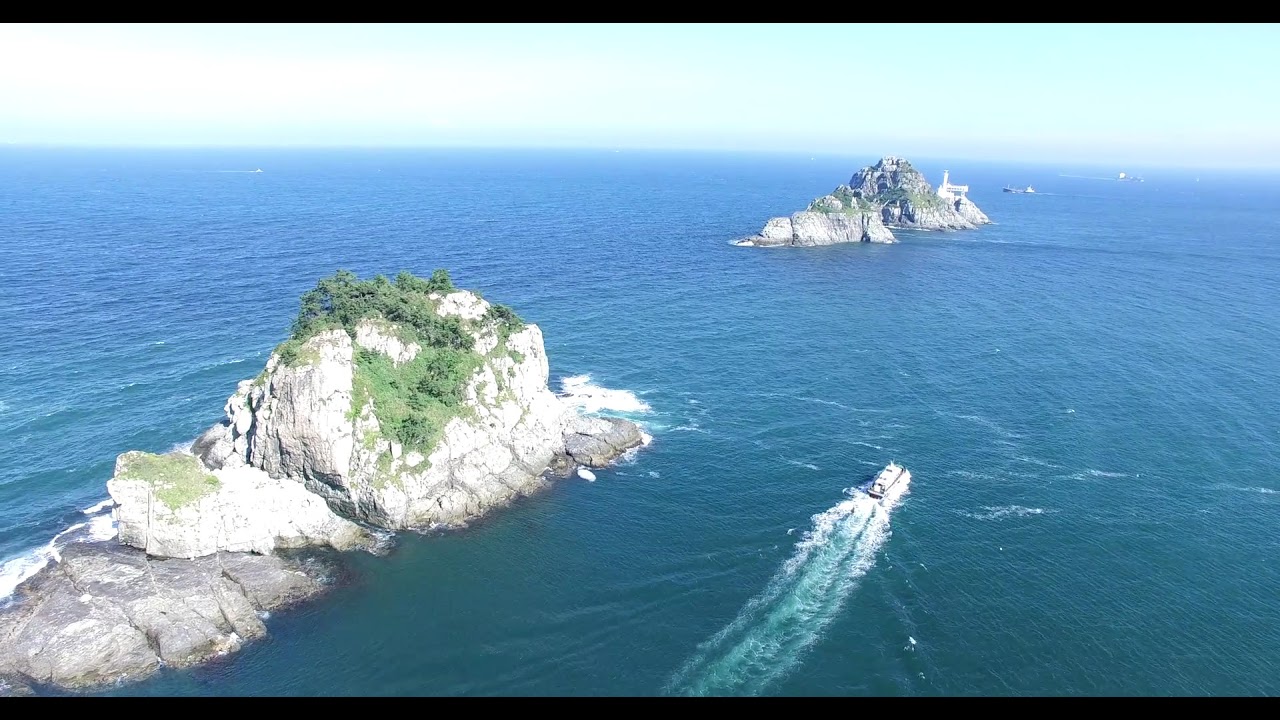The image showcases an ocean scene with two small rock formations or islands, adorned with sparse vegetation and some trees, rising out of the bright aqua blue water. The formations are relatively close together, roughly a hundred boat lengths apart. In the foreground, to the right of the nearer rock formation, a boat speeds by, leaving a visible white wake behind it. On the horizon, a couple more boats can be seen, appearing small due to the distance. The sky above is a pale, nearly shiny white, possibly with some light cloud coverage on the left side. The overall composition of the image is wide, resembling the format of a high-definition television screen, and it is framed by narrow black bars at the top and bottom.